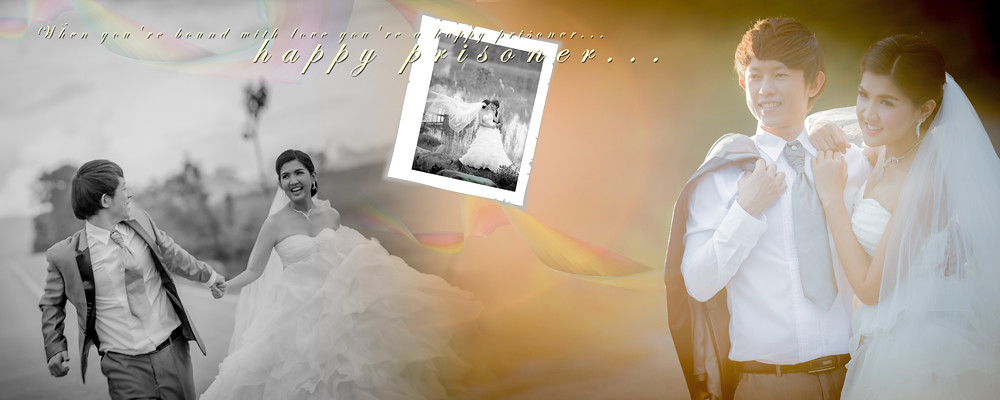This evocative image presents a multi-layered narrative of love and togetherness, intriguingly blending past and present. In the upper left corner against a gradient background transitioning from gray to light brown, an inscription reads: "When you're bound with love, you're a happy pioneer." Below this message, in larger white letters, the phrase "Happy Prisoner" stands out prominently.

On the lower left side, a captivating scene unfolds: a smiling wedding couple gazing lovingly at each other as they walk forward. The man looks dapper in a classic tuxedo and tie, while the woman radiates joy in a voluminous white wedding dress. The exact colors are unclear, adding a timeless quality to the image.

Contrasting this, the right side of the picture takes us back in time with an endearing photograph of the same couple as children. The boy is adorably dressed in a brown suit, and the girl wears a mini wedding dress, capturing the innocence of their childhood dreams.

At the center of the composition, a small postage stamp-sized photo, slightly tilted, provides another glimpse of the couple, though details are less discernible. The clever juxtaposition of these images beautifully illustrates the enduring bond and journey of this loving pair from their youthful imaginations to their real-life union.